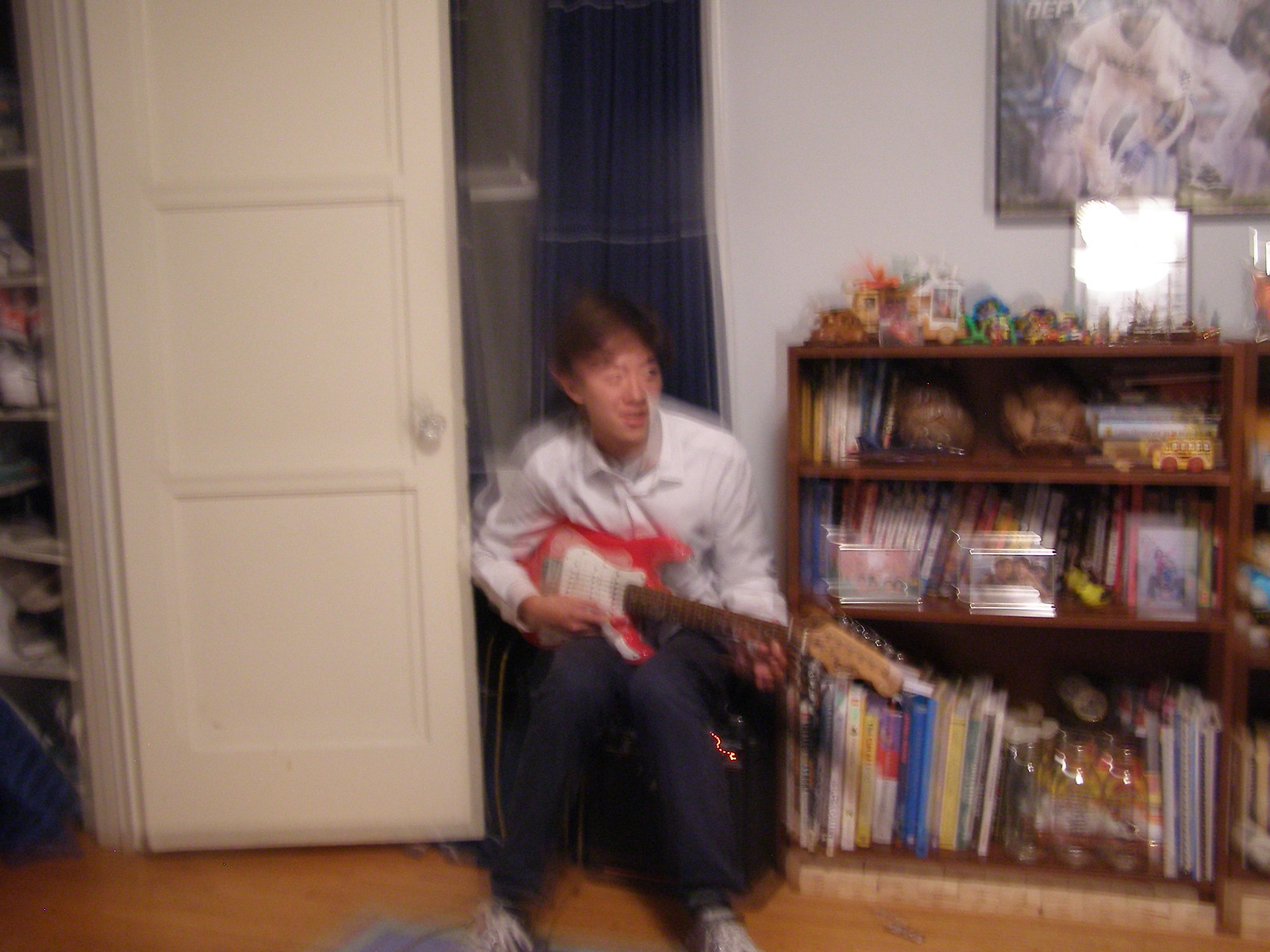A person is captured playing a bright red guitar with a brown handle, seated on what appears to be a wooden box, possibly functioning as an amplifier. The scene is set in a cozy bedroom, where the individual sits beside a bookshelf brimming with books, small toys, and various figurines adorning the top shelf. The room features a gray-colored wall with a painting hanging on it and a blue curtain partially visible. A white door leads to a closet that displays an assortment of sneakers. The hardwood floor is partially covered by a small corner of a carpet. The guitarist, dressed in sneakers, jeans, and a dress shirt, seems to be performing solo, perhaps during a quiet moment at a house party or in the comfort of their own home.